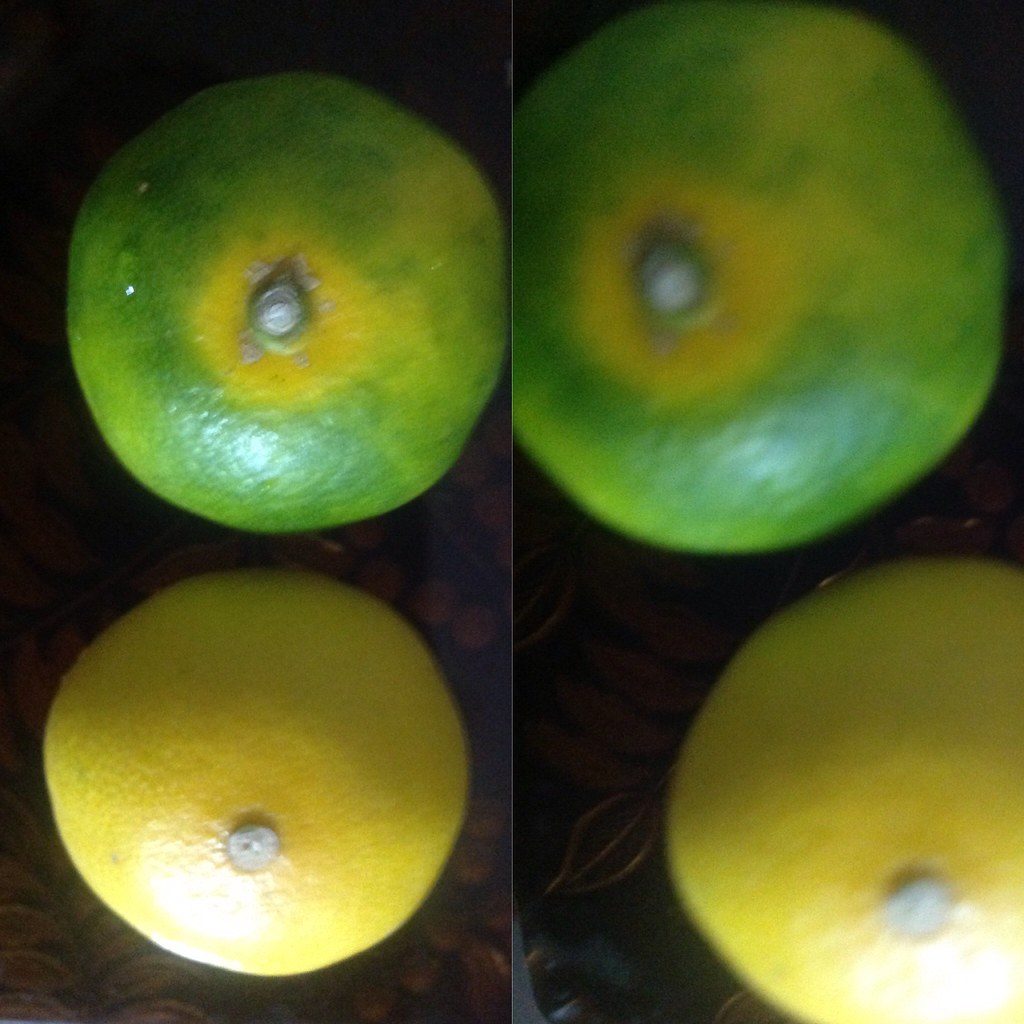In this side-by-side composition, two photographs showcase a lime and a lemon positioned similarly in both images. The upper fruit is a lime featuring green skin with yellowish blotches indicative of aging or over-ripening, while the lower fruit is a fully ripened, bright yellow lemon. Both fruits are displayed stem-up against a dark, indeterminate background. The photo on the left is relatively clearer, though still somewhat out of focus, whereas the photo on the right is a closer, more blurred, and off-center version of the same scene, with parts of the lime and lemon cut off at the top and bottom edges, respectively. A bit of white flash or light is visible on the bottom side of the lemon in the darker context of both images.